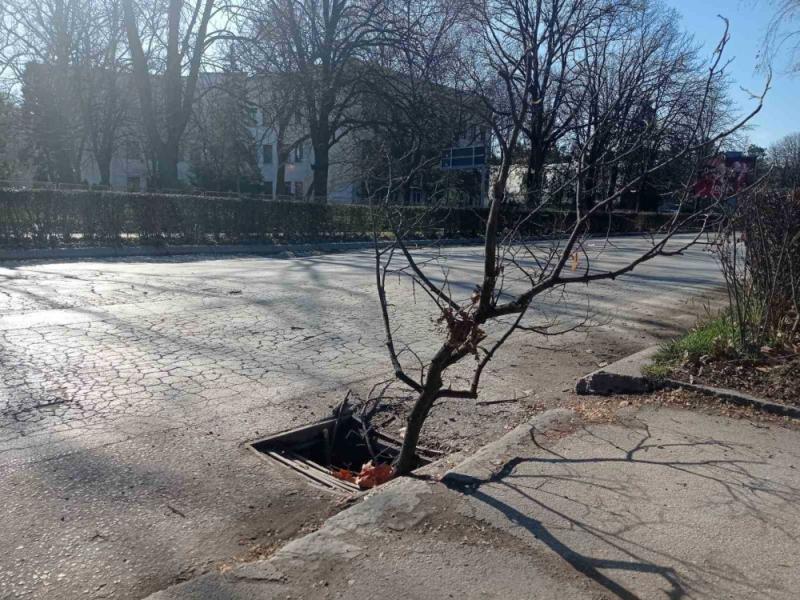The image depicts a deserted, deteriorating street with noticeable cracks forming intricate patterns across the gray pavement. The road is seen from the perspective of someone standing on a sidewalk or driveway entryway. Dominating the foreground is a broken roadside grate positioned near the curb, from which a large, dead tree branch with multiple skinny limbs protrudes, giving the impression of the tree bursting through the grate. A large sycamore leaf rests near the trunk. To the side is a small patch of green grass, while the background shows a line of brown, leafless hedges separating the road from a three-story white building. The surroundings hint at a winter scene, with all trees devoid of foliage. The overall image lacks any signs of human activity, emphasizing the desolation of the scene.